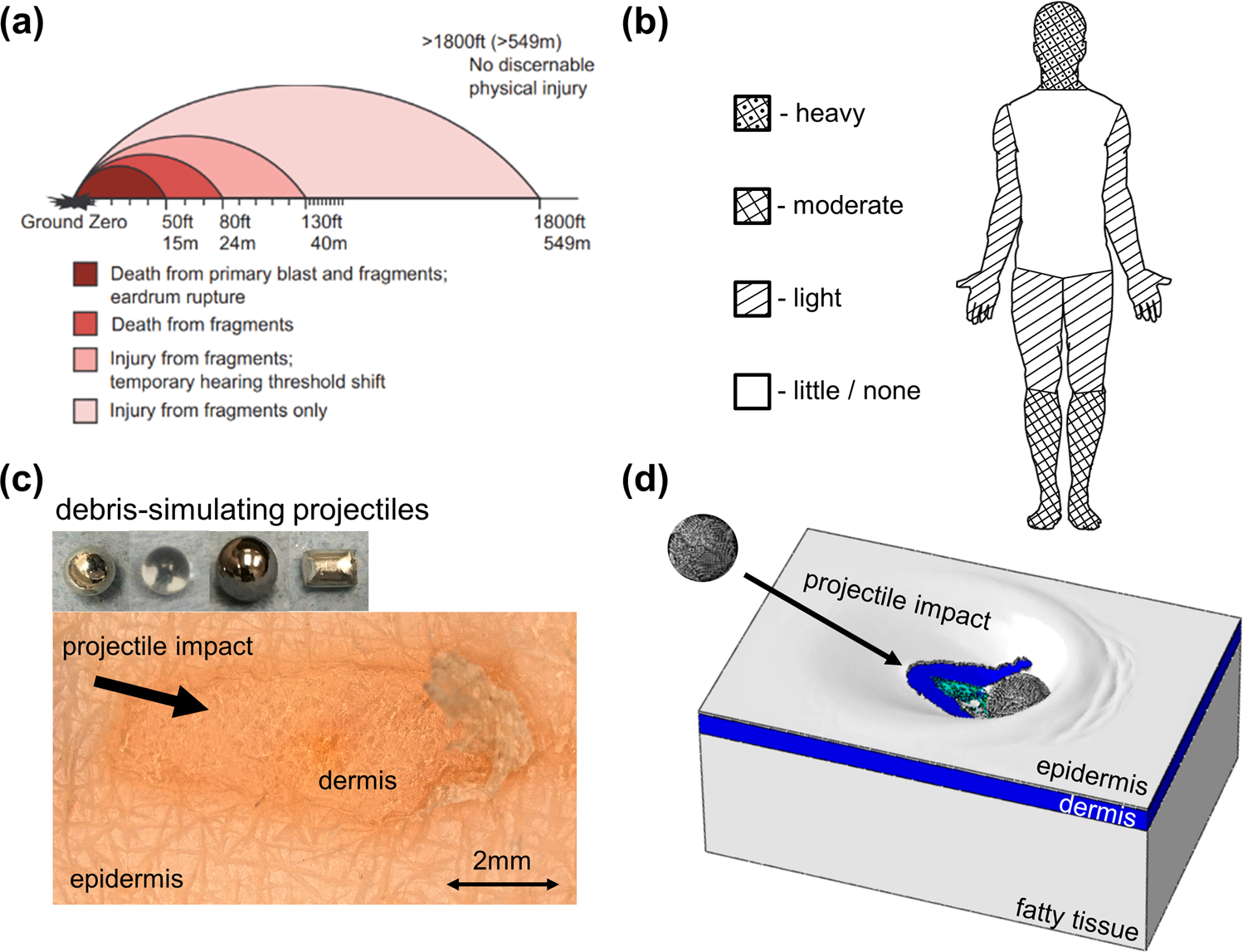The image is a detailed screenshot from a textbook displaying the damaging effects of various types of bombs, including pipe bombs loaded with metal objects, on the human body and skin. At the top left, there is a primary diagram labeled 'A,' depicting an oval-shaped graph with colored zones indicating the range of impact—from ground zero in purple, progressing through red (50 to 80 feet), pink (80 to 130 feet), to tan (130 to 1,800 feet). This diagram is accompanied by a key explaining the levels of damage: death from primary blast and fragments, and injuries from fragments. Below it, 'B'  presents a rear view of a human figure marked with zones illustrating levels of injury from heavy to none. Additional sections 'C' and 'D' include diagrams of debris simulating projectiles and a detailed view of projectile impact on fatty tissue and 2mm of epidermis.